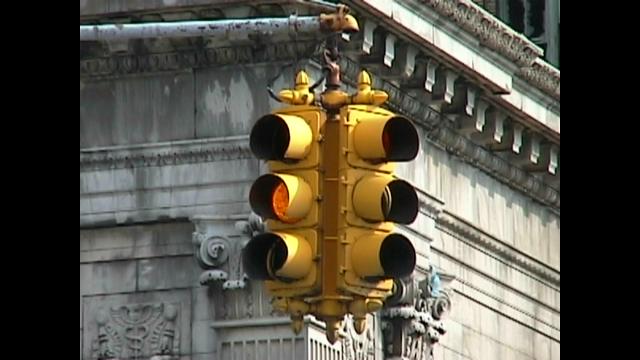The photograph captures a close-up view of a yellow streetlight set against a stone building characterized by its intricate detailing and a mixture of light and dark grey hues. The streetlight, suspended from a thick, somewhat weathered silver metal rod, features a light housing with multiple yellow lights, including one illuminated in the middle to indicate caution or yield. This building, potentially a historical courthouse or church, showcases a lot of architectural carvings, including pillars, embroidery resembling the medical symbol, and ornate patterns that frame the streetlight. The image is taken during daylight, as evidenced by the natural light illuminating the scene. In the background, another taller concrete building is visible, adding depth to the backdrop of this detailed and carefully composed photograph.